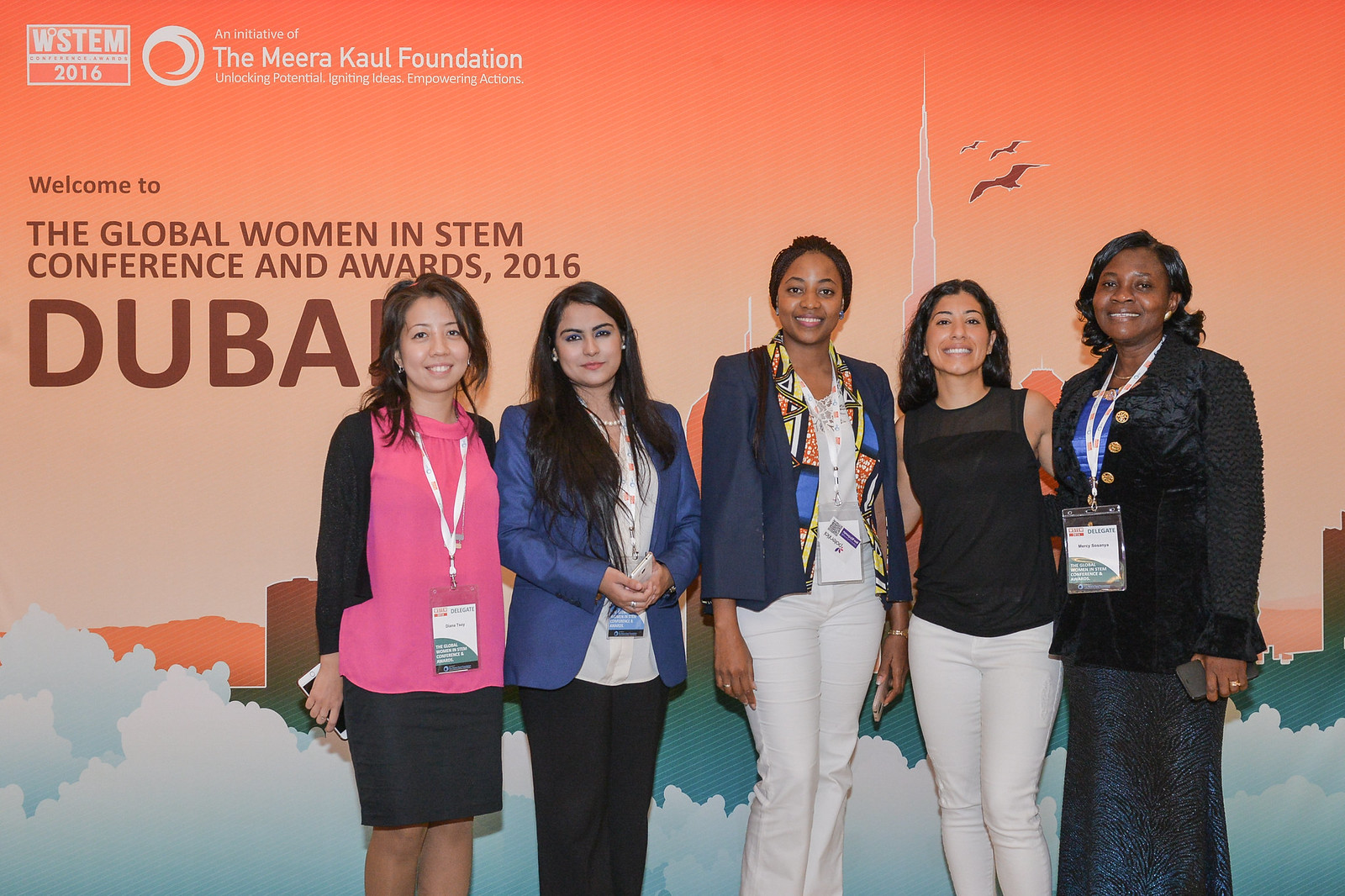Five women are standing in front of a large conference poster with an orange and red gradient background that resembles a sunrise or sunset. The bottom of the poster has a depiction of clouds, giving a dreamy appearance, with silhouettes of Dubai's skyline, including a tall, white tower. At the top left of the poster, in white letters, it reads "WSTEM 2016," followed by a circle logo. Below this, in dark brown letters, it states "Welcome to the Global Women in STEM Conference and Awards 2016, Dubai." Next to this, in white letters, is the name "Meera Kaul Foundation."

The five women appear to be of diverse ethnic backgrounds, including Asian, Indian, and African-American. They are a mix of formal and casual outfits. One woman wears a sleeveless dark top, another is dressed in a blue blazer over a white shirt, while another has a pink and black top paired with a gray knee-length skirt. The fourth woman is in white pants with a blue shirt, and the fifth, who appears older, is in a black sweater and dress with a prominent lanyard.

All five women are smiling and holding identification lanyards, looking confidently at the camera, embodying the spirit of the Global Women in STEM event.